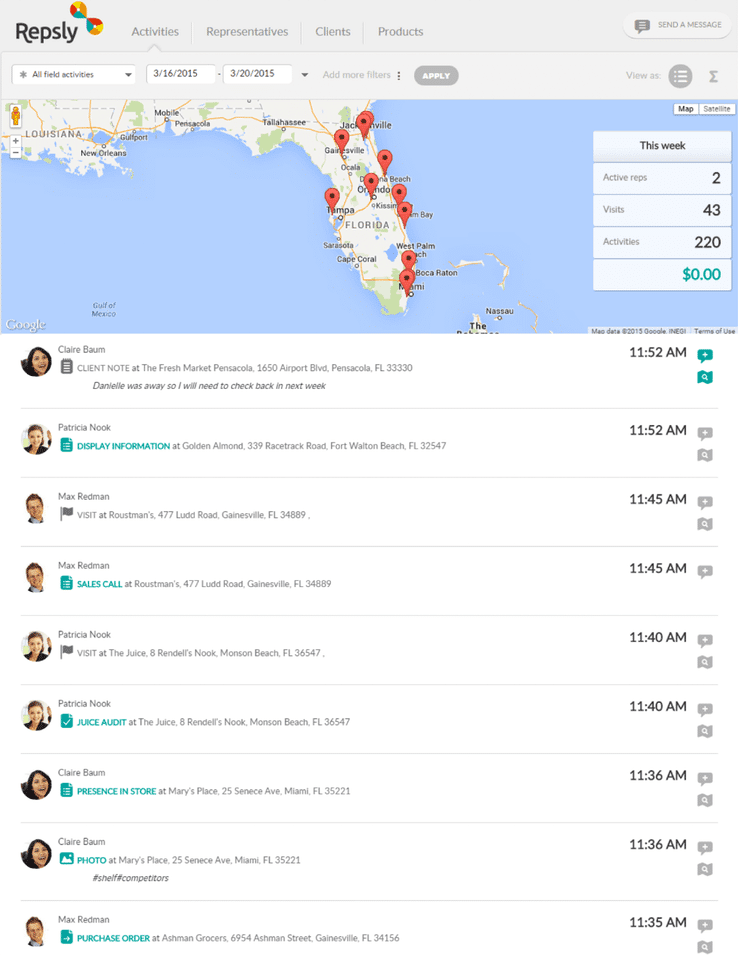This vertical screenshot captures an interface from the Repsly application. The light gray header bar at the top features the bold black text "Repsly" in the upper-left corner, accompanied by a colorful icon. The navigation menu includes options for Activities, Representatives, Clients, and Products. At the top-right corner, there is a "Send a Message" button. Directly below the header, the interface displays three horizontal white text boxes. The first box is labeled "All Field Activities," the second box shows the date range "3-16-2015," and the third box displays the date "3-20-2015." Additional icons are present on this navigation bar for various functions.

Below the navigation bar lies a detailed map of Florida, accentuated by the surrounding ocean. The map features several highlighted red location icons. To the right of the map, a labeled box titled "This Week" displays numerical data. Underneath the map, there are multiple white horizontal columns. Each column starts with a profile picture on the left side, followed by the corresponding name and small light gray text. To the right of each column, there are time stamps indicating the activities, all of which occurred in the morning. The top time stamp is flanked by two highlighted green icons, while the rest of the time stamps down the column feature gray icons.